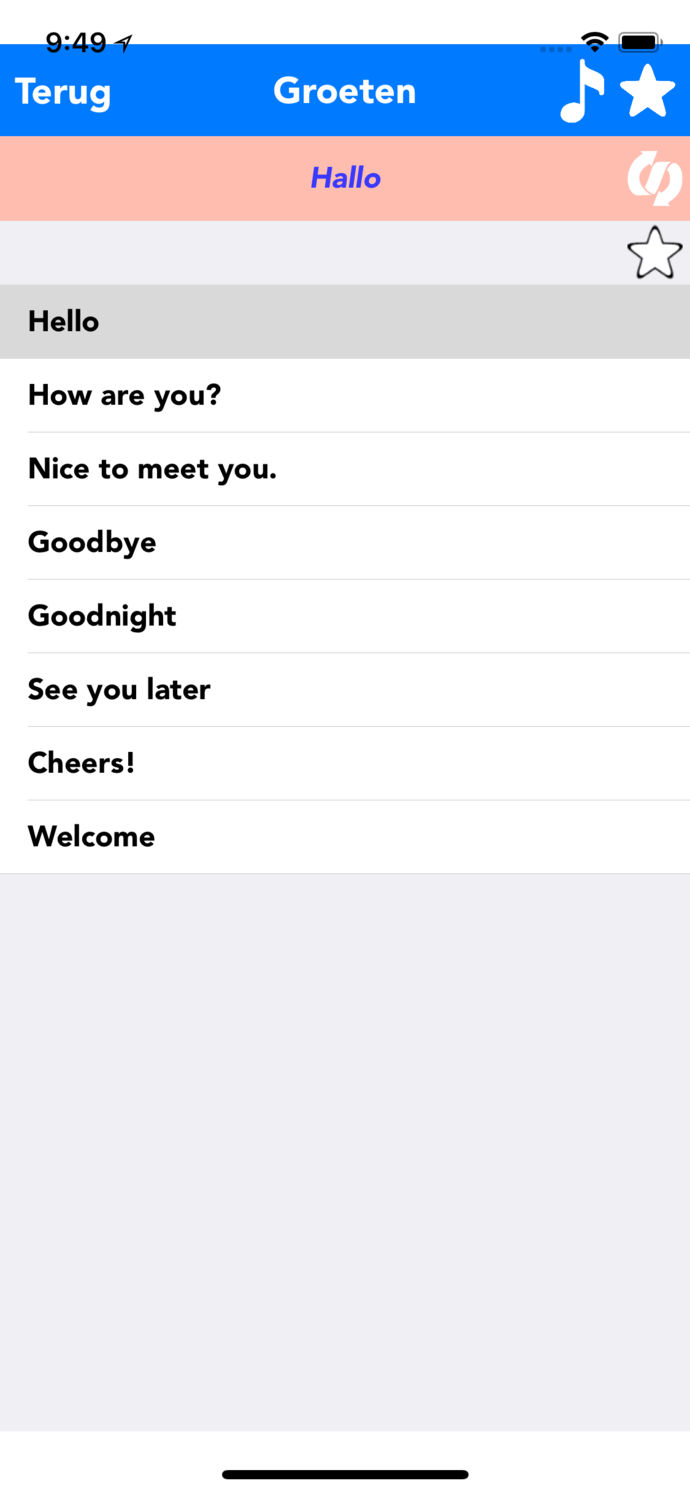The image displays a tablet or phone screen. At the top of the screen, there is a status bar showing the time "9:49," the Wi-Fi signal strength, and the battery level. The top section has a blue background overlaid on a black bar that provides device information.

Centrally positioned in the blue bar is the word "Groeten" (capitalized as G-R-O-E-T-E-N). On the left side of this blue section, the word "Terug" (capitalized as T-E-R-U-G) is displayed, and on the right side, there are icons of a musical note and a star.

Below the blue bar, a pink bar features the word "Hallo" (H-A-L-L-O) in blue text. Beneath this pink bar, there is a star icon followed by the text: "Hello, how are you, nice to meet you, goodbye, goodnight, see you later, cheers, and welcome."

Further down, there is a large blank box shaded in lilac, and beneath this box, there is a prominent black line. Additionally, next to the word "Hallo" in the pink bar, there is an "S" character that appears to be tipped on its side.